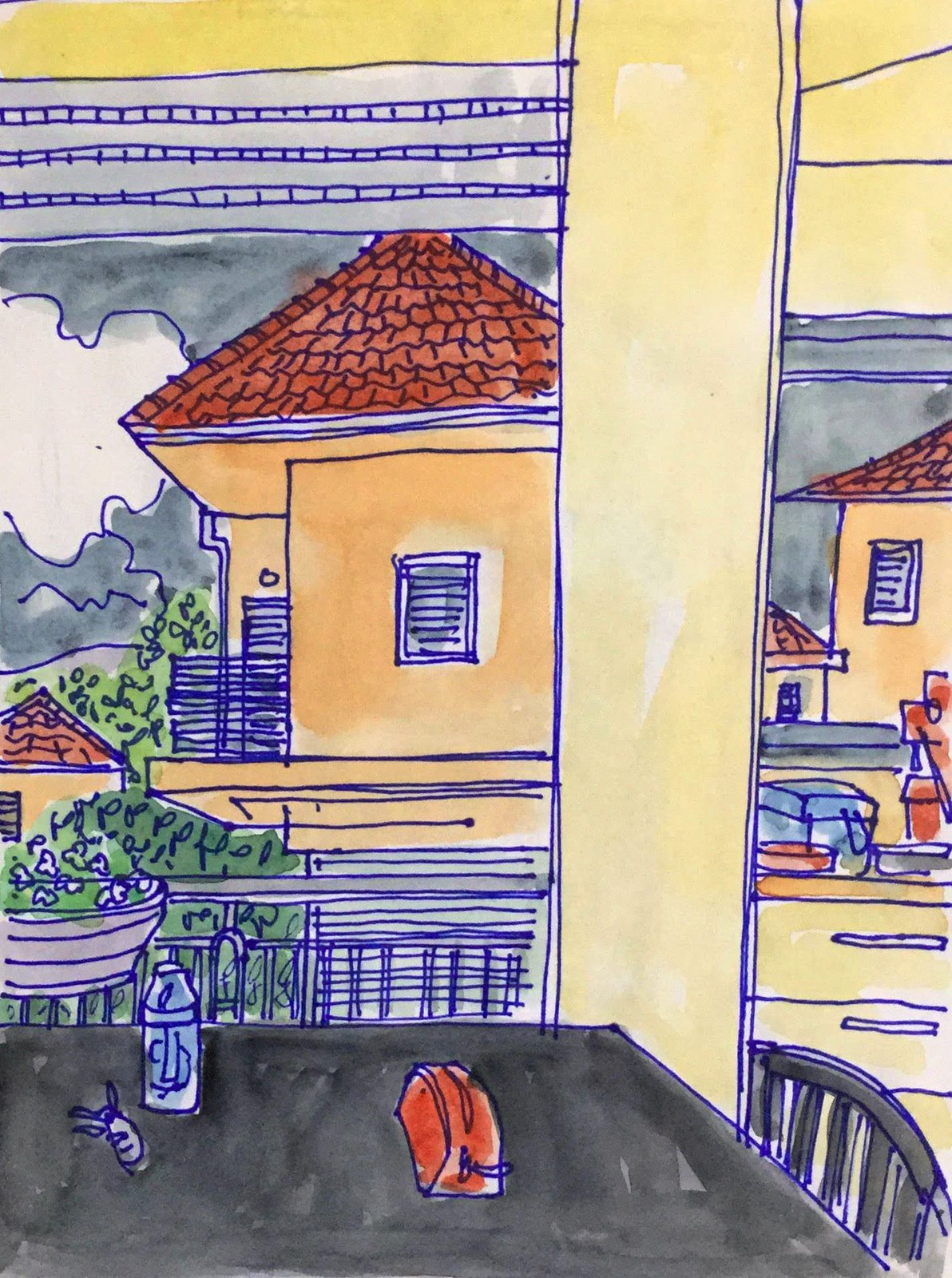The image is a detailed hand-drawn artwork, likely created by a beginner or a child, executed with blue pen and accented with watercolor. It depicts a scene that appears to be either a kitchen or a porch, with a view extending out through large windows or openings onto a street. In the foreground, there is a dark gray dining table featuring various items: a water bottle, what might be a dead fish, a plate, a basket, a pot, a toaster, and an object resembling an orange purse or eyeglasses case. Adjacent to the table is a chair, and nearby are several drawers or other kitchen furniture.

Through the windows or slats, the view outside reveals light orange or terracotta-style buildings with balconies, adorned with red roofs, and framed by trees and bushes. There are at least four houses or apartments visible, each with distinct features like windows and potentially a patio supported by a yellow beam. The sky above is decorated with clouds, contributing to the impression of an expansive, outdoor scene. Additionally, a railing with a potted plant can be spotted in the background, adding to the intricate detail of this artwork.